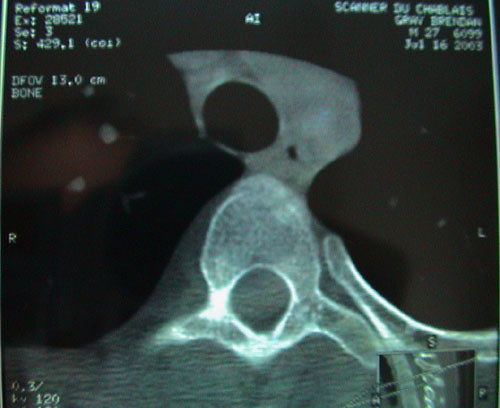This image appears to be a rectangular, almost square photograph of an x-ray featuring a black background typical of x-ray imagery. The central focus shows illuminated portions that seem to be bones, though it's unclear which specific bones are depicted. In the center, the brightest part of the image reveals structures that resemble curved handles converging into an oval shape with a central void. Additionally, another bone extends downward to the right, connected to various smaller bones. In the upper left corner, there is printed data including "19" and "EX2002, set 3, S429.1, DFOV 13.0 cm, bone." The upper right corner holds more information, potentially the patient's name and date of birth, alongside the word "scanner." Notably, the top center of the image displays the text "AI." The bottom right corner hints at a shoulder structure, further adding to the details captured in this x-ray photograph.